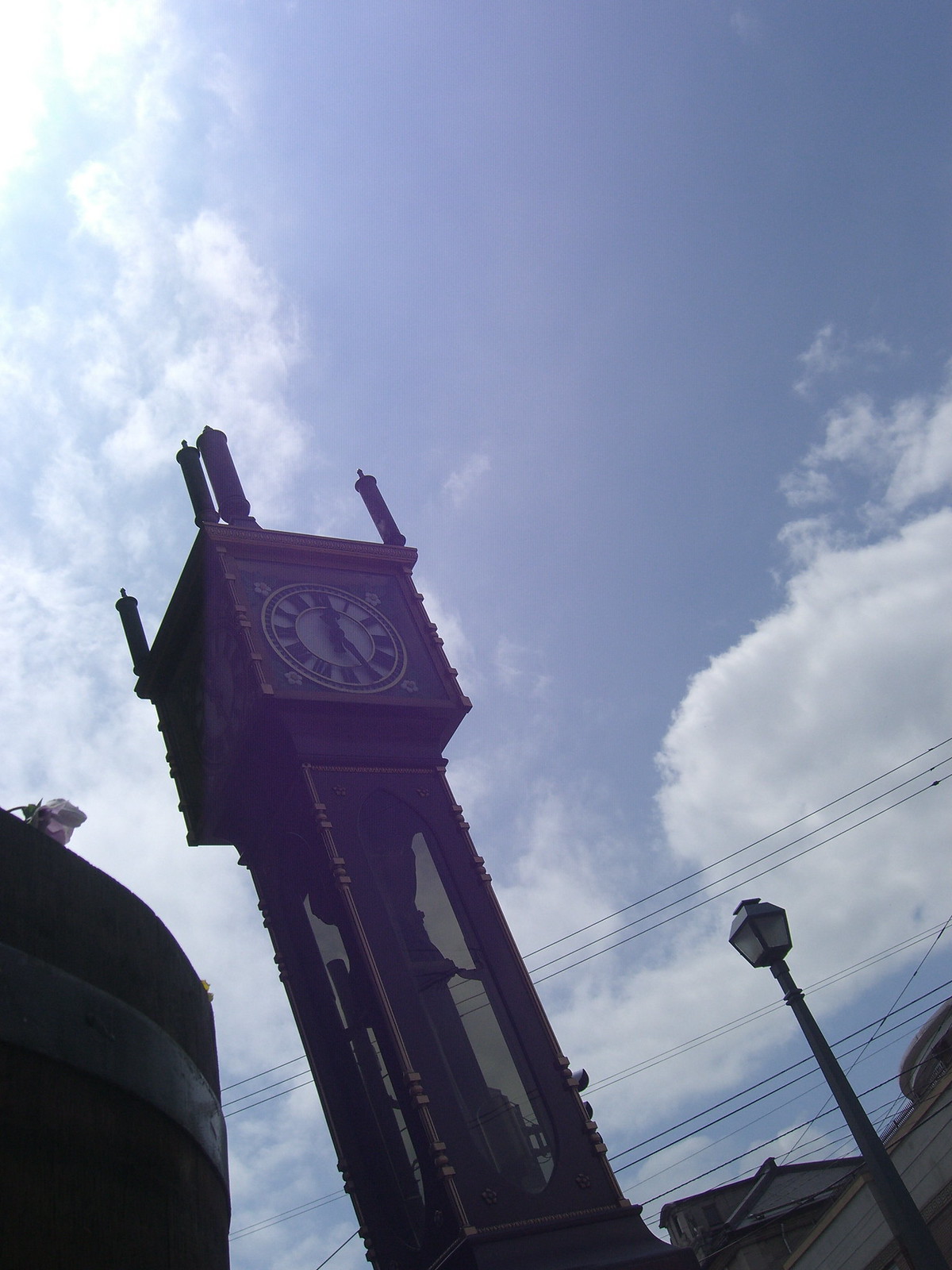The photograph captures a striking tall clock tower situated prominently in a town square. The tower, constructed from sturdy brown wood, features glass panes that offer a peek through, revealing glimpses of the skyline. The design suggests a pendulum-style clock, though the internal mechanics are obscured from view. Photographed from a corner angle, the wood structure partially frames a brilliant blue sky adorned with fluffy white clouds.

In the lower section of the image, a small black lamppost can be seen to the right, adding a touch of quaint charm, while a rustic brown whiskey barrel sits to the left. At the summit of the tower rests a square wooden clock, displaying faces on all four sides. Each clock face is white and marked with black Roman numerals from I to XII, standing out boldly against the structure. This scene offers a harmonious blend of classic timekeeping and picturesque town square elements set against a serene sky.